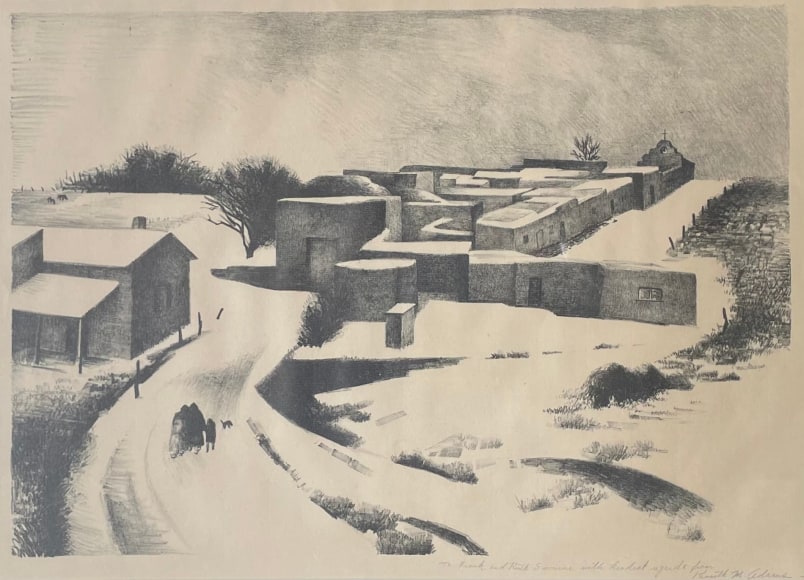This black and white pencil or charcoal drawing captures a serene snow-covered scene, reminiscent of a quaint Spanish or Mexican village. The composition features a road that winds from the lower left corner towards the center, bisecting a landscape blanketed in snow. On the left middle of the picture stands a solitary house, while in the center lies a cluster of attached, stone-built houses with snow-covered rooftops. The background reveals a sparse forest, with leafless trees poking out, particularly noticeable in the upper left and right corners. On the right side, dead trees or short winter-dormant bushes add to the wintry ambiance. Behind the cluster of houses, and slightly to the right, agricultural land extends, hinting at the village's rural character. Far in the distance, a church stands as a focal point, anchoring the peaceful village in its winter shroud.